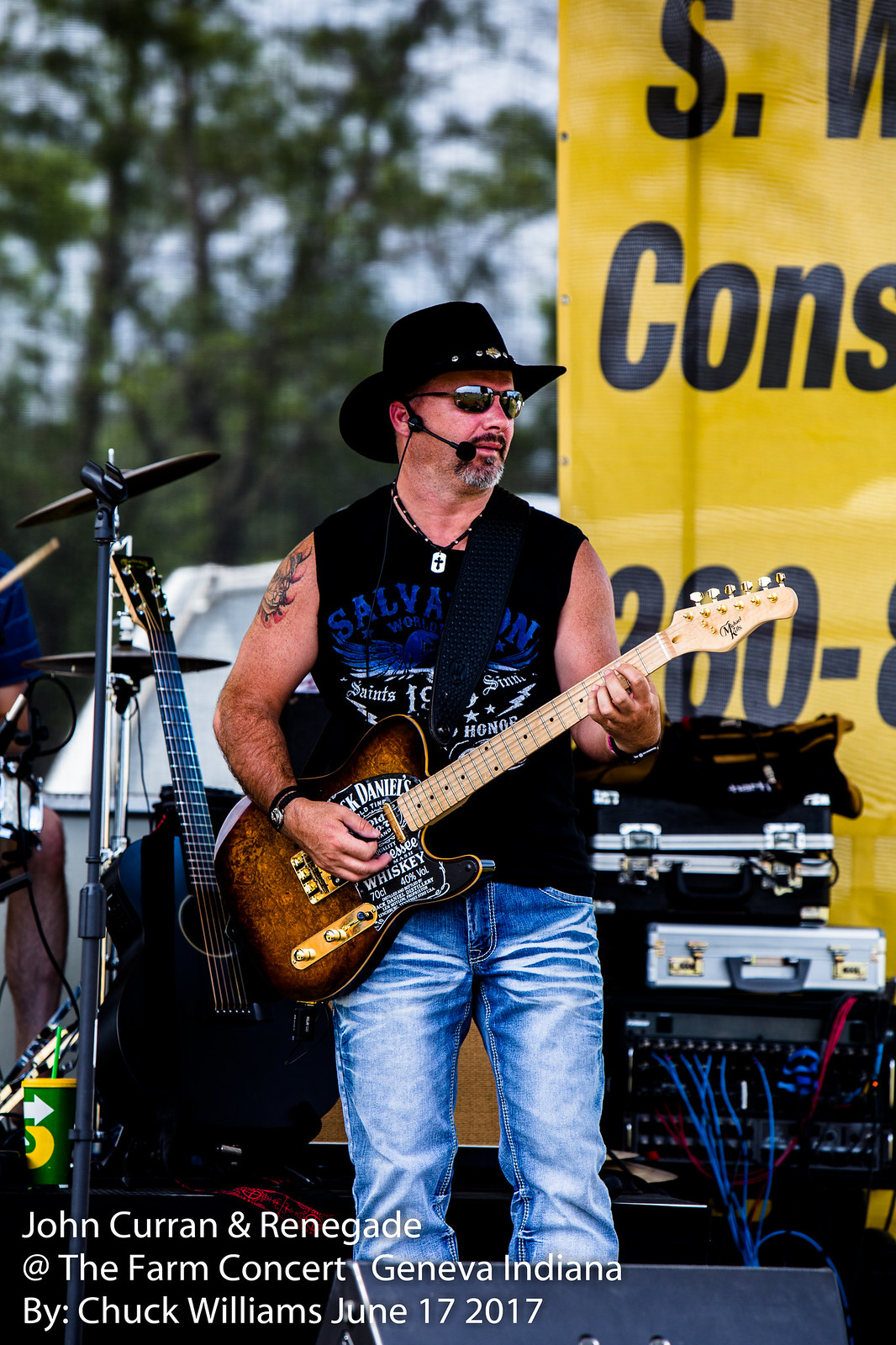In the image, a man is passionately playing an electric guitar on stage at an outdoor concert during the day. Dressed in blue jeans and a black and blue sleeveless t-shirt, he draws attention with his cowboy hat, sunglasses, and an earpiece microphone. The man, standing upright from his ankles to the top of his head, is positioned centrally towards the bottom of this vertical photograph. A distinctive tattoo marks his right shoulder as he grips a brown and black guitar, adorned with a Jack Daniels liquor logo on its pickboard and a light brown wooden neck. 

Behind him, musical equipment and a yellow backdrop with obscured black text occupy the stage. Trees are visible on the left side, adding a touch of nature to the setting. To his right, a guitar rests in its stand, and parts of a drum kit are also visible, hinting at the presence of a full band. The atmosphere radiates vibrant colors including yellow, black, beige, brown, blue, silver, white, and dark green. 

Adding a personal touch, white text in the bottom left corner reads, "John Curran and Renegade at The Farm Concert, Geneva, Indiana by Chuck Williams, June 17, 2017," contextualizing the lively scene captured in this photograph.